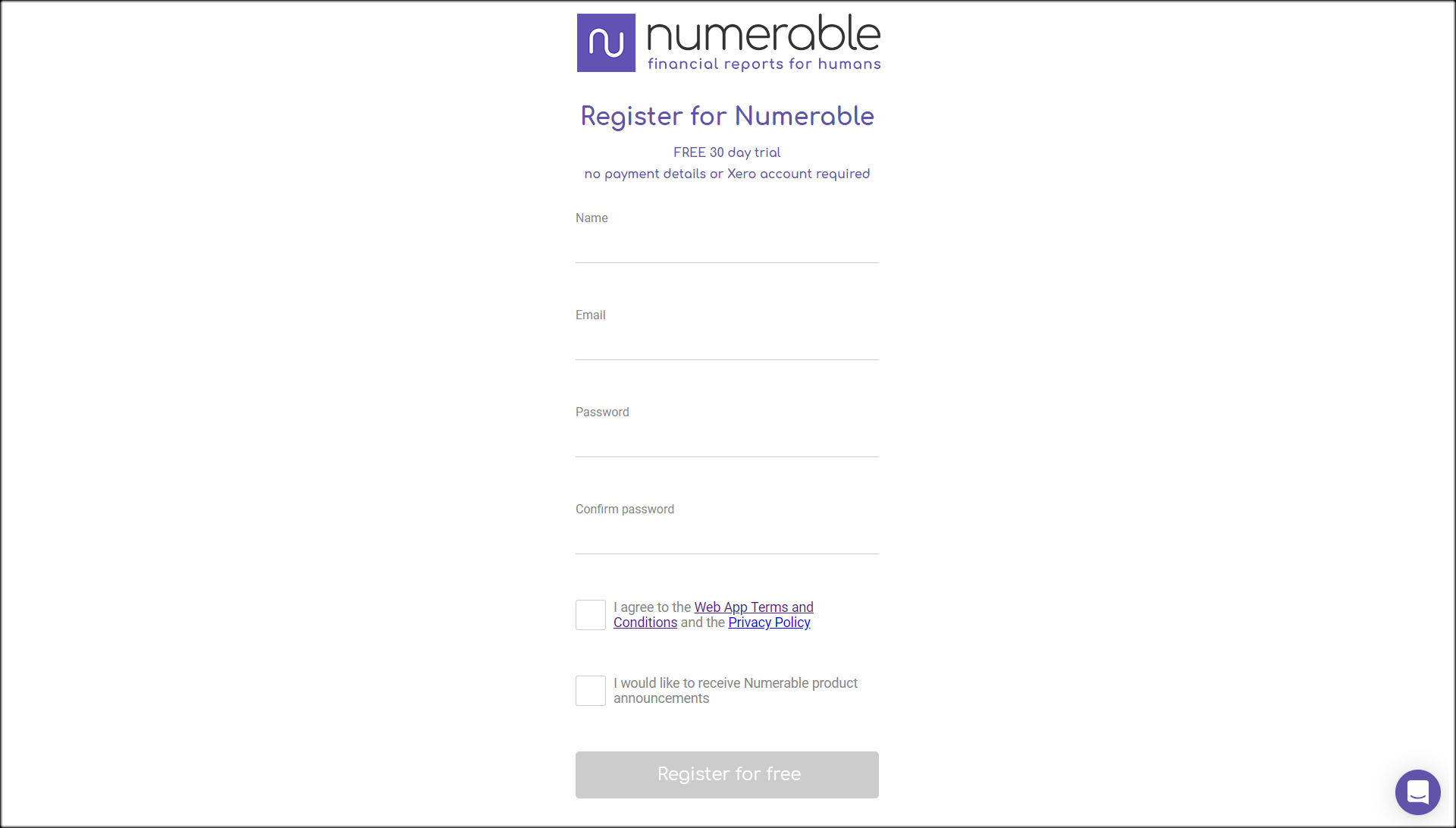The image is a vertical screenshot from a mobile device or app, displaying a registration page titled "Numerable: Financial Reports for Humans." At the top, it features the Numerable logo—a stylized, squiggly depiction of the letters "N" and "U" inside a purple square. Below the logo, the text "Register for Numerable" is displayed in a purple font, followed by a smaller purple font note stating, "Free 30-day trial, no payment details required."

The page includes greyed-out fields for entering a name, email, password, and password confirmation. Below these fields are two unchecked boxes; the first one is labeled "I agree to web app terms and conditions and the privacy policy," with "terms and conditions" linked in purple and "privacy policy" linked in blue, indicating that users can click these to view more details. The second checkbox states, "I would like to receive Numerable product announcements."

At the bottom, the "Register for Free" button is also greyed out, indicating that the form cannot be submitted until all required information is entered and the checkboxes are selected. In the bottom-right corner, there is a chat logo, suggesting that users can click it to ask questions or seek assistance.